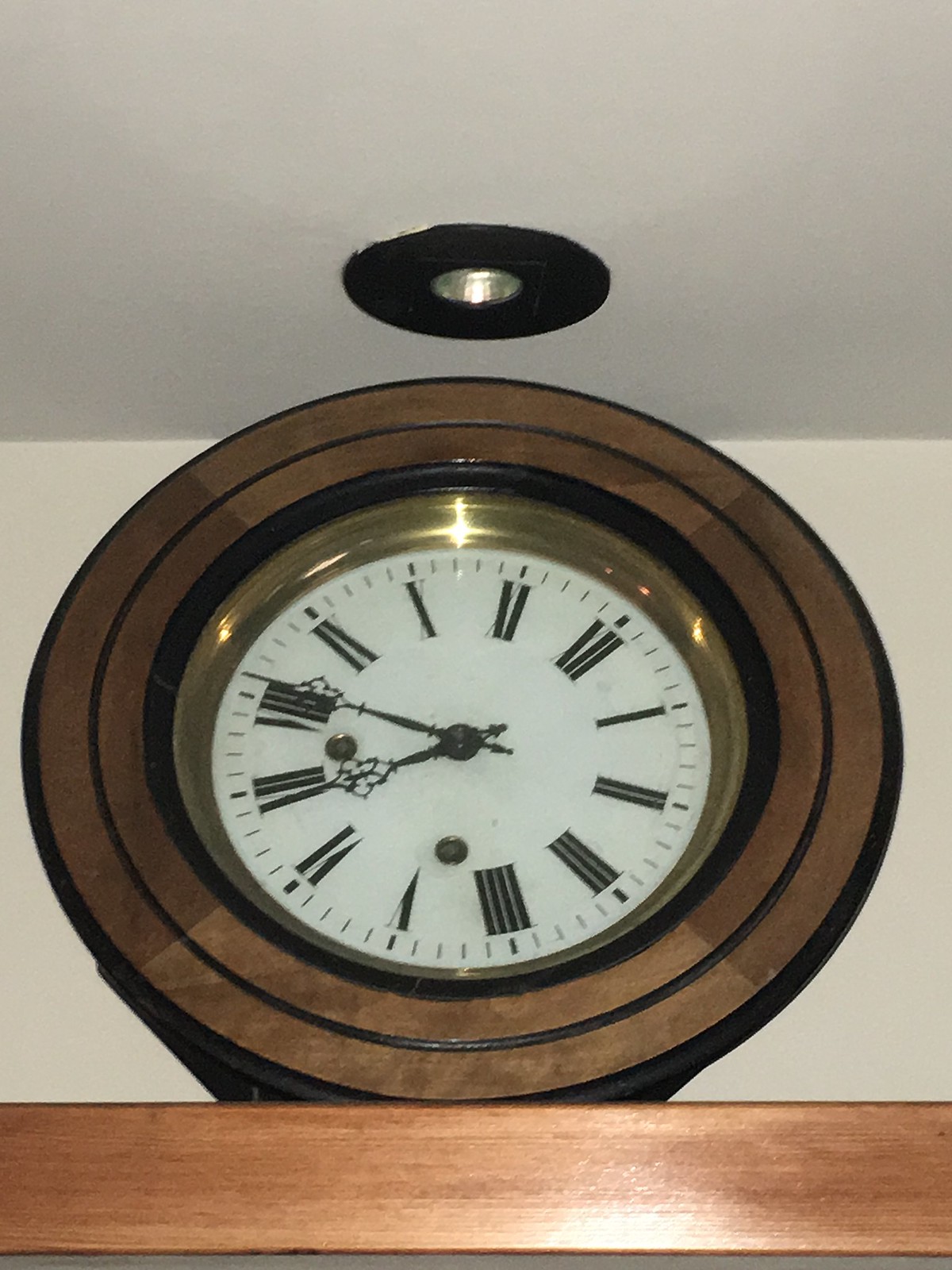This detailed photograph captures a round analog clock prominently displayed on a wooden shelf. The background is evenly split between a white ceiling and the upper part of a white wall, featuring a recessed spotlight near the ceiling. The clock, which is not aligned straight up, features Roman numerals from I to XII, black minute markers, and black hands that indicate the time as 6:42. Its design includes a white clock face, surrounded by a gold rim and encased in an elegant, possibly mahogany, brown wooden frame with intricate inlay work. The wooden shelf spans the width of the image, reinforcing the clock's placement on it rather than being wall-mounted.